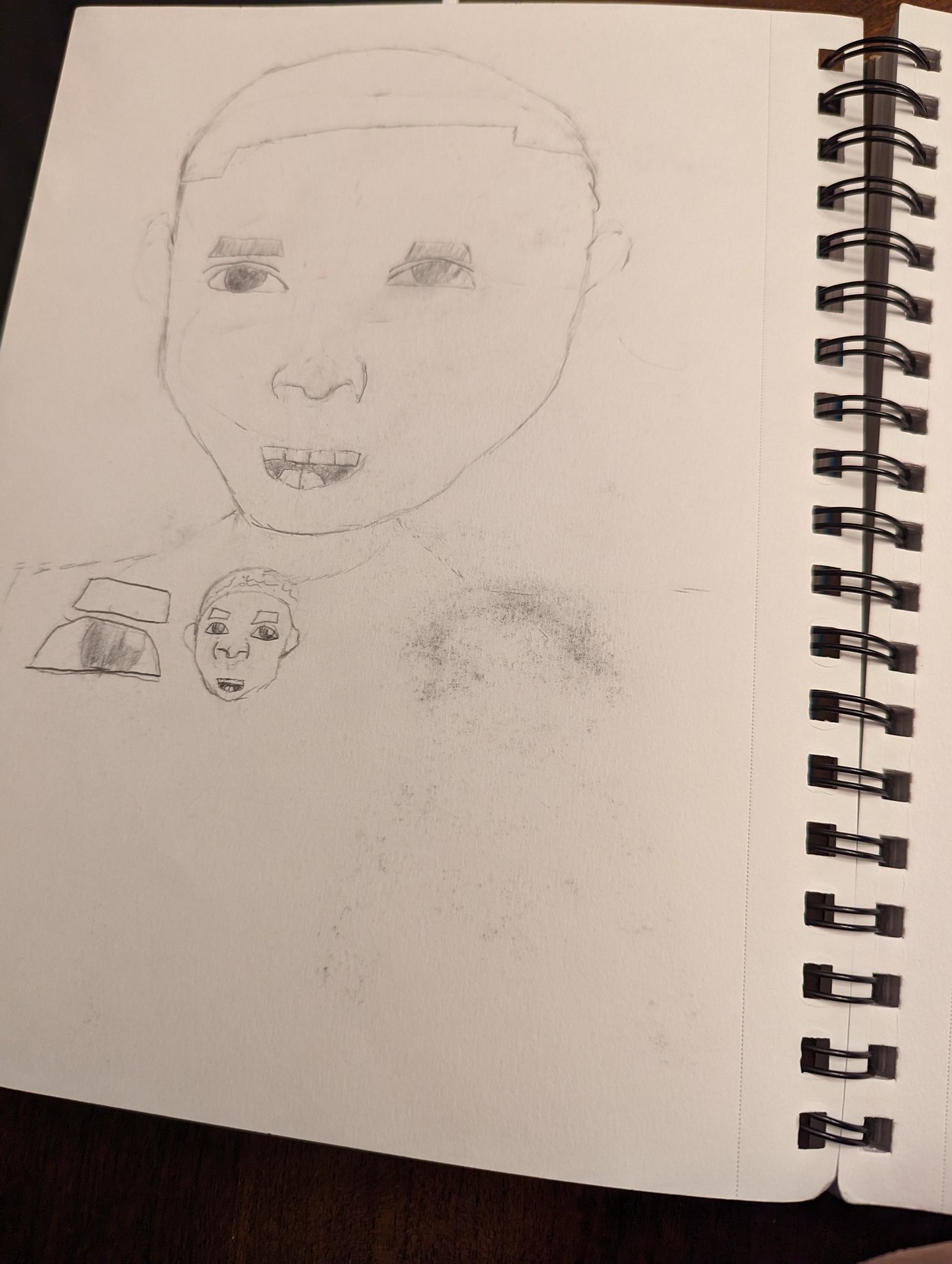The image appears to be a detailed sketch from a sketchbook, presented on white paper. The sketchbook is bound on the right side with a colorful binding, featuring rings that loop through holes along the edge of the pages. 

The primary focus of the drawing is a boy with a distinct hairstyle resembling a bowl cut. His facial features are detailed, showcasing trapezoidal eyebrows and a wide-eyed expression. His nose is clearly defined, and his mouth is open, revealing four upper teeth and his tongue. 

The boy's neck transitions down to his shoulders, which are drawn in a straightforward manner. 

In the lower-left corner of the drawing, there is a depiction of black people, and above this section, a large rectangle dominates the top part of the sketch. Nearby, there is also a smaller face that appears similar to the main figure, though with some proportional differences. 

Additionally, there is a noticeable smudge of black ink on the right side of the page, adding an element of texture and imperfection to the overall composition.